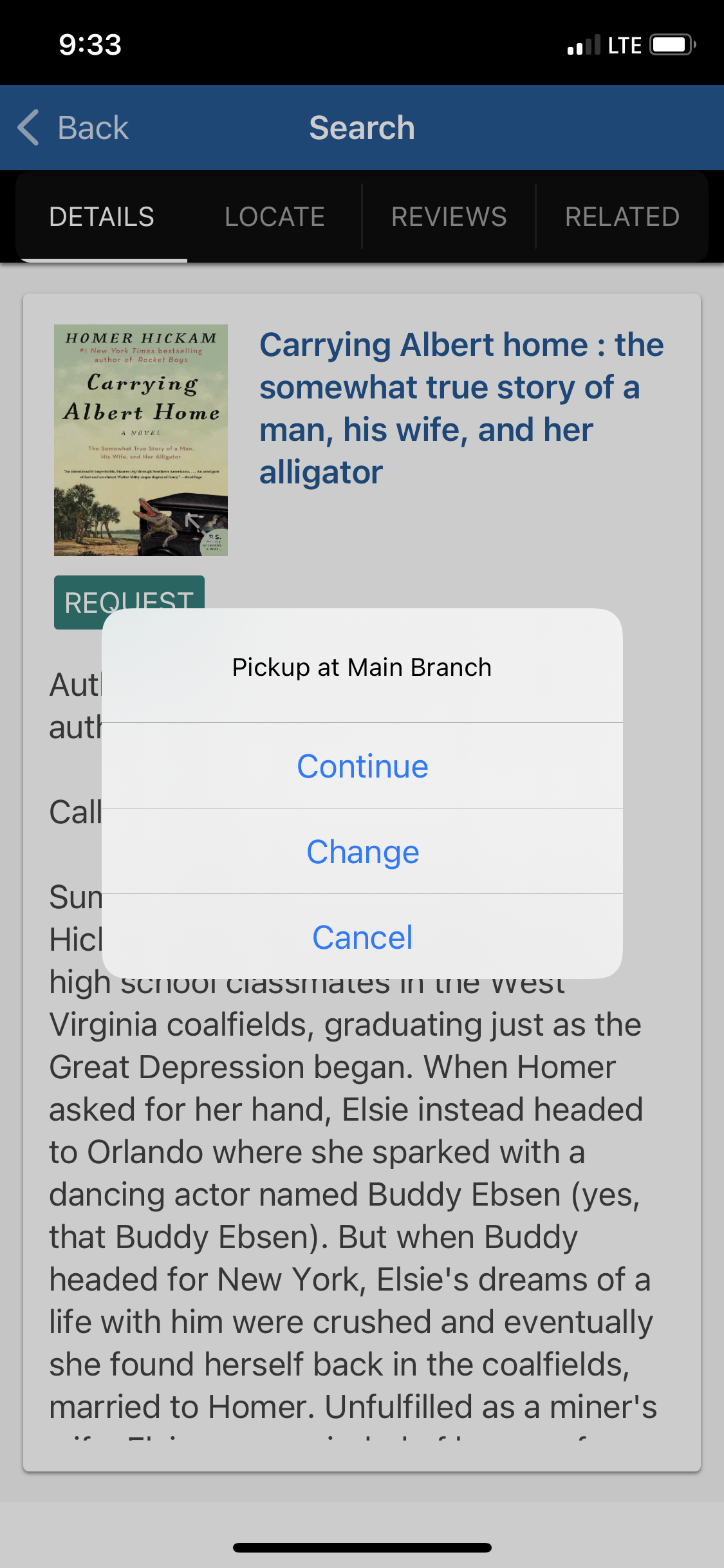At the very top of the screen, the background is black, displaying the time as 9:33 in the corner. To the right, a horizontal battery icon is nearly full, followed by the letters LTE, indicating a strong network connection. Below this, a long blue rectangle centers the word "Search," underneath which an arrow pointing left and the word "Back" are situated on the left side.

Directly below this toolbar, the word "Details" is underlined, followed to the right by "Locate," "Reviews," and "Related." Descending further, an image of a book cover is prominently displayed. The cover features a picturesque scene with sand, water, and a tree in the background, against a bluish-gray backdrop. The book title, “Carrying Albert Home,” is clearly visible on the cover.

To the right of the book image, in blue text, it reads, "Carrying Albert Home: The Somewhat True Story of a Man, His Wife, and Her Alligator." Adjacent to this, there is a white box, which at its top states, "Pick up at Main Branch." Below this, in blue text, options are presented: "Continue," followed by a line beneath, along with "Change" and "Cancel."

Directly below these options is a synopsis of the book, provided in black text.